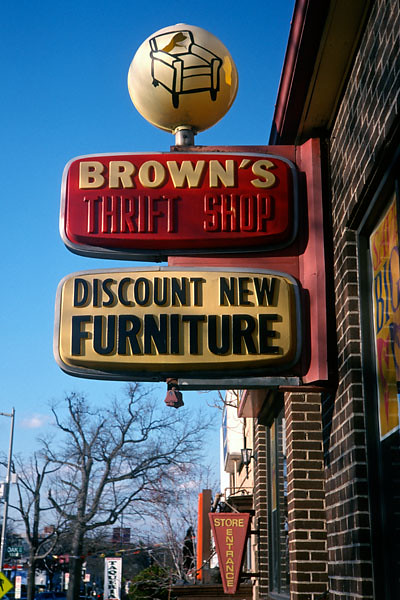The image features an array of signs displayed outside a shop located at the top of the street. The topmost sign showcases an illustration of a reclining chair or seat, hinting at the nature of the store's offerings. Directly below this, a prominent red sign with white text reads "Browns Thrift Shop," while the words "Thrift Shop" are inscribed in red, providing a striking contrast. Just beneath this, a white sign with bold black lettering announces "Discount New Furniture," suggesting bargain deals on fresh, unused items. In the background, another sign indicating "Store Entrance" is partially visible, guiding potential customers towards the entry point of the establishment.